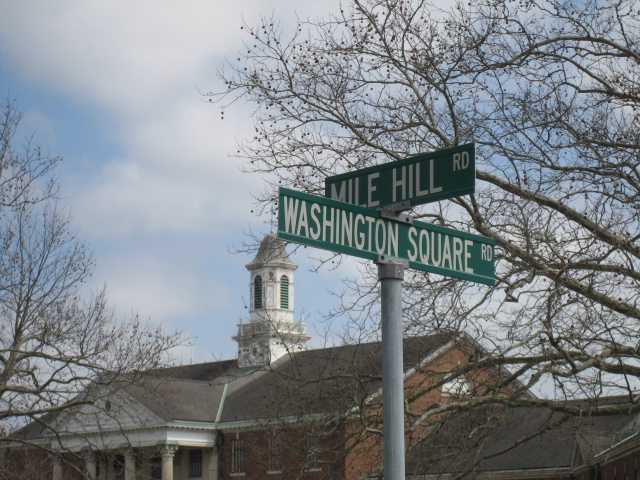In this detailed photograph, the viewer is presented with a striking image of a street sign at the intersection of Mile Hill Road and Washington Square Road. The street signs are rectangular and green with white lettering, mounted on a tall metal post. The perspective of the shot is from below the signs, making them a prominent feature in the foreground. 

Behind the street signs, two large, leafless trees stand starkly against the pale blue sky, which is dotted with white clouds, suggesting the cold bareness of winter. The absence of leaves casts a distinct seasonal atmosphere over the scene, amplifying the chill of what appears to be either autumn or winter.

Dominating the background is a grand red brick building characterized by its ornate architecture. The structure boasts a large awning-type area at its front, accentuated by four imposing white pillars. Atop this historic building sits a white structure, possibly a bell tower or lookout tower, indicating its significance and grandeur. This architectural style hints that the building could be a university, courthouse, municipal building, school, or even a hospital, although its exact purpose remains open to interpretation. The combination of these elements creates a scene rich in historical and seasonal context.